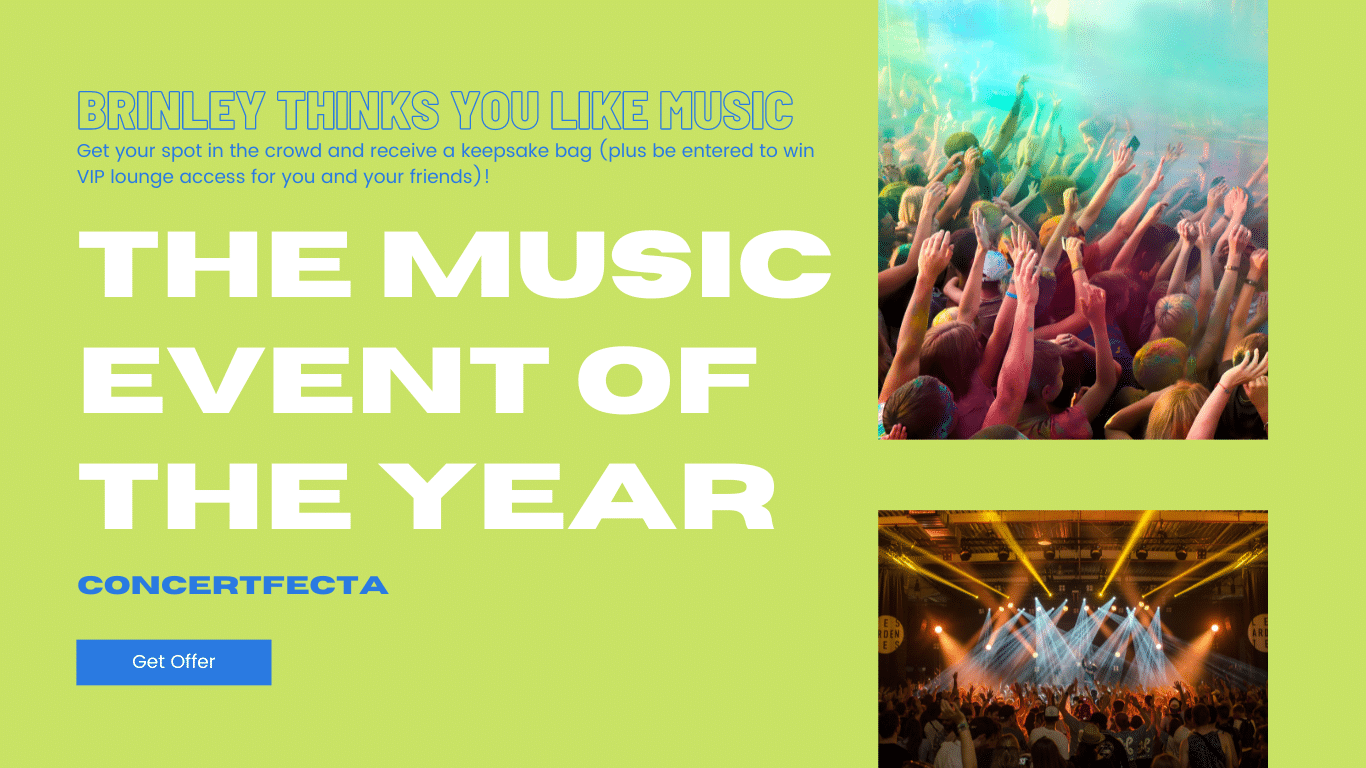In this promotional image for the music event of the year, the background is a vibrant lime green. At the top left, a welcoming message reads, "Brinley thinks you like music. Get your spot in the crowd and receive a keepsake bag, plus be entered to win VIP lounge access for you and your friends!" in an engaging and enthusiastic tone. 

Centered in bold white capital letters, the heading announces: "THE MUSIC EVENT OF THE YEAR." Directly below, in a striking blue font, the event is named "Concert Fecta." Further down, a prominent blue box with white text encourages viewers to "Get Offer."

On the right side of the image, there are two photographs. The top photo depicts a lively concert scene, crowded with fans tightly packed together. Many are holding up their cell phones or waving their hands in the air, capturing the electric atmosphere. The bottom photo provides a wider shot, showcasing the dynamic lighting as beams cascade down onto the energized audience below, highlighting the magnitude and excitement of the event.